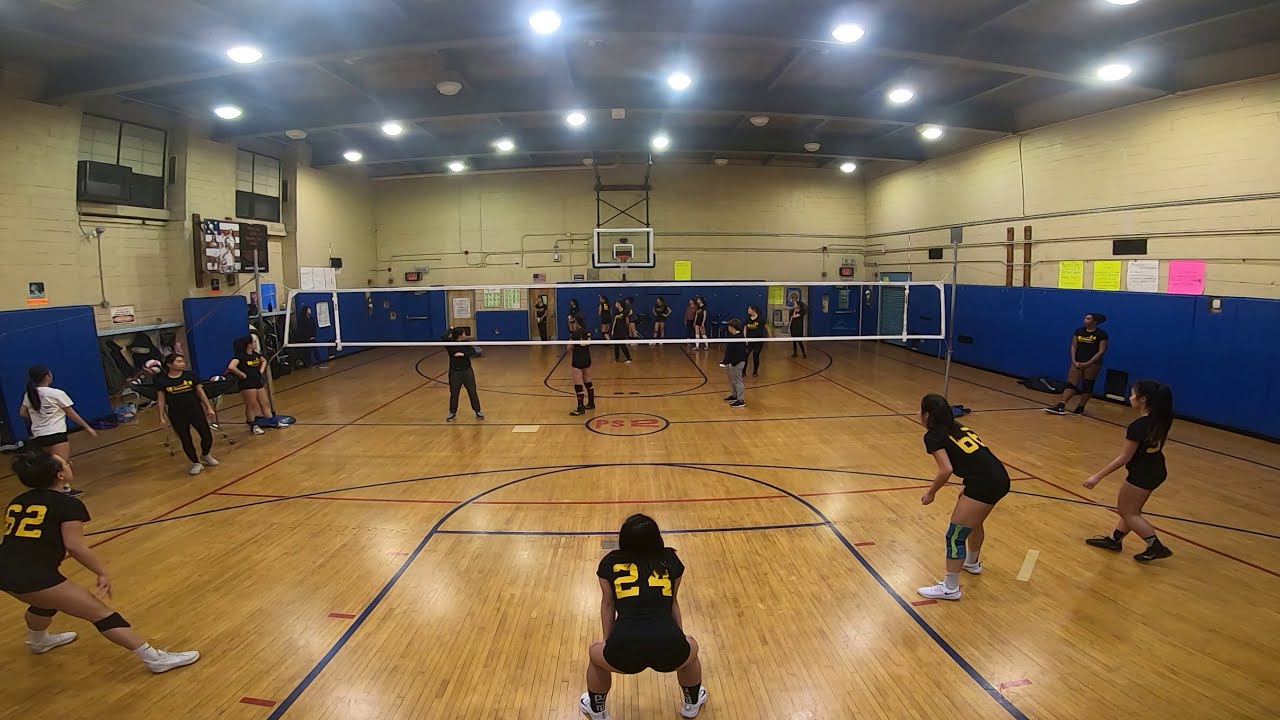In this image, an indoor gymnasium is captured during what appears to be a practice session of a girls' volleyball game. The gym features a shared basketball and volleyball court, distinguished by red and blue tape markings on the floor. A white and black volleyball net is prominently stretched across the center of the court. In the foreground, four girls from one team, wearing black jerseys with yellow numbers and matching volleyball shorts, knee pads, and sneakers, are positioned in a ready stance with bent knees and hands on their knees. The girl at the very bottom center of the image sports the number 24 on her back. The gymnasium is well-lit with a grid-style ceiling and various overhead lights. Blue padded mats line the walls, alongside yellow, white, and pink poster boards, and visible conduits. To the far back, there are more girls from the opposing team and several people along the wall, possibly coaches or other team members. A basketball hoop hangs from the ceiling, underscoring the multi-purpose nature of the gym. An air conditioner is mounted in one of the windows, contributing to the indoor environment. This detailed scene captures the energy and preparation typical of a volleyball practice.